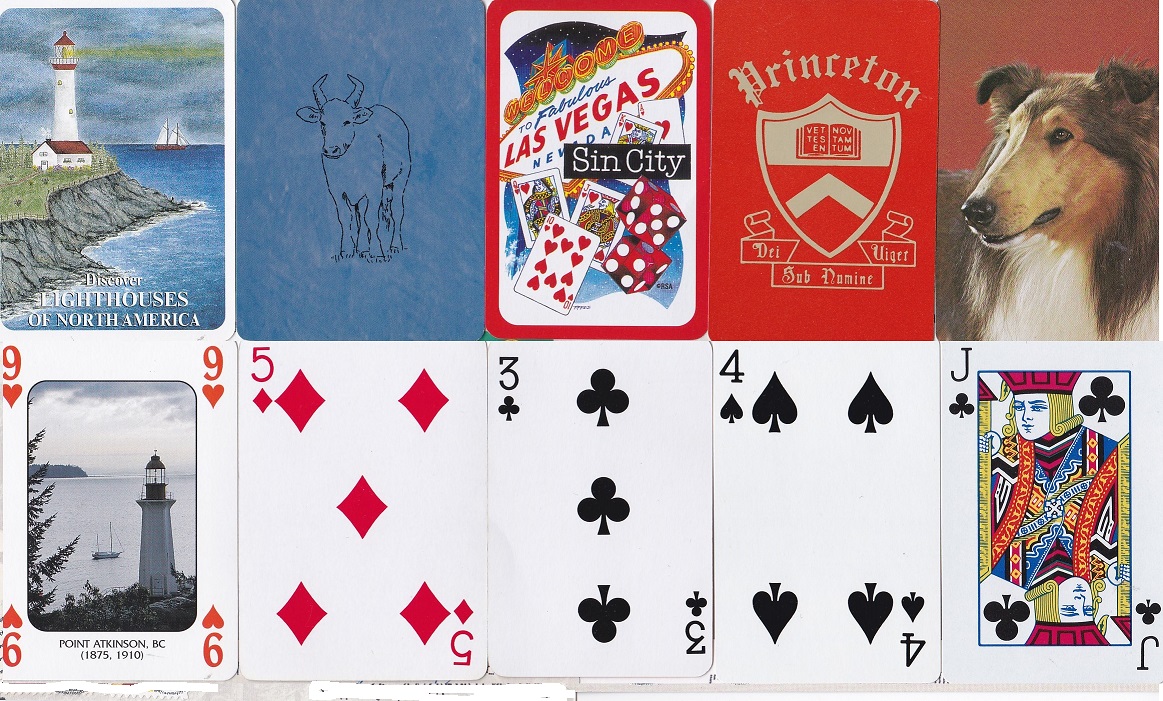In this collection, we have an array of playing cards showcasing both their fronts and backs, each portraying unique and vivid scenes. 

The first card features a picturesque lighthouse setting from "Lighthouses of North America." The scene is awash with a blue, cloudy sky under which a sailboat glides serenely on the water. The lighthouse, a towering white structure with a red top, stands prominently on the shore, accompanied by a smaller white house, also capped in red. Below this captivating image is the nine of hearts, displaying a small white lighthouse and a sailboat.

The second card presents a minimalistic yet striking design. It is a blue card featuring the outline of a ram in black ink. Underneath this illustration is the five of diamonds.

Next in the series is a card celebrating Las Vegas, often dubbed "Sin City." This card highlights the iconic Las Vegas sign in red and white, with "Sin City" inscribed in a black square with white lettering. The imagery includes classic casino symbols such as cards and dice, and below it lies the three of clubs.

A card from Princeton University follows, showcasing a red background with silver print. The design includes Princeton’s prestigious coat of arms in red and silver hues. Accompanying this emblem is the four of spades.

The final card in the set pays homage to Lassie, the beloved collie. Set against a bold red background, Lassie is depicted with her characteristic brown face accented by black and white fur. The card is completed by the jack of clubs.

Each card in this group offers a detailed and vibrant snapshot, blending artistry with the timeless charm of playing cards.